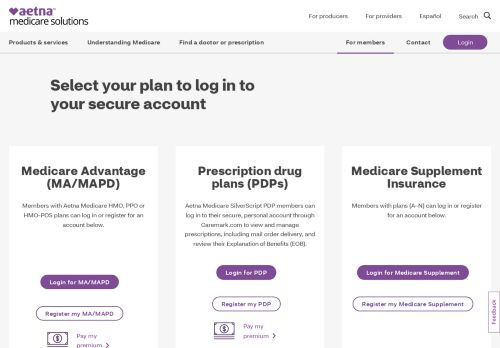This website screenshot for Aetna features the company's branding prominently displayed in the upper left-hand corner. The Aetna logo, which includes a purple heart followed by the word "Aetna" in lowercase purple letters, sets a welcoming tone. Directly below the logo, the text "Medicare Solutions" appears in black lowercase letters.

Beneath this, a navigation menu spans the top of the image. While a bit blurry, the menu items from left to right include "Medics and Services," "Understanding Medicare," "Find a Doctor or Prescriptions," and "For Members," which is underlined in purple, indicating the current section. Additional menu options include "Contact" and a purple lozenge-shaped button labeled "Login" in white text.

The header underneath the menu instructs, "Select your plan to log into your secure account." Below this header, a grid layout displays three white boxes from left to right. Each box represents a different plan option:

1. **Medicare Advantage (MA/MAPD)**: This box contains a brief description of Medicare Advantage plans, followed by “Login” and “Register” icons.
2. **Prescription Drug Plans (PDPs)**: In the center, this box offers information on Prescription Drug Plans, also accompanied by “Login” and “Register” icons.
3. **Medicare Supplement Insurance**: The right-hand box provides details on Medicare Supplement Insurance, with the similar “Login” and “Register” options.

Each section gives users clear and concise options to either login or register, tailored to their specific Medicare plan needs.